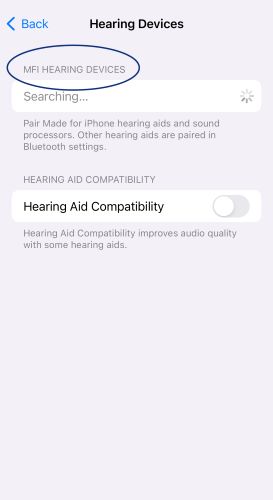The image is a screenshot from an iPhone, designed to help users pair and manage MFi (Made for iPhone) hearing devices. At the top of the screenshot, there is a navigation bar with a back button on the top left, featuring a blue arrow and the word "Back" in blue text. The title "Hearing Devices" is prominently displayed in black text at the very top, followed by "MFi Hearing Devices" enclosed within a teal-colored oval.

Beneath this, there is a section with a small box that shows the status "Searching..." along with an animation indicating that the device is actively looking for available hearing aids. Below this section, there is instructional text that reads, "Pair Made for iPhone hearing aids and sound processors. Other hearing aids are paired in Bluetooth settings."

Further down, there is a section labeled "Hearing Aid Compatibility," which includes a toggle switch. Instructions beneath this switch explain that enabling hearing aid compatibility can improve audio quality with some hearing aids. The overall design of the interface features a clean layout with grey and black text on a white and off-white background, giving it the appearance of a standard instructional panel on a smartphone.